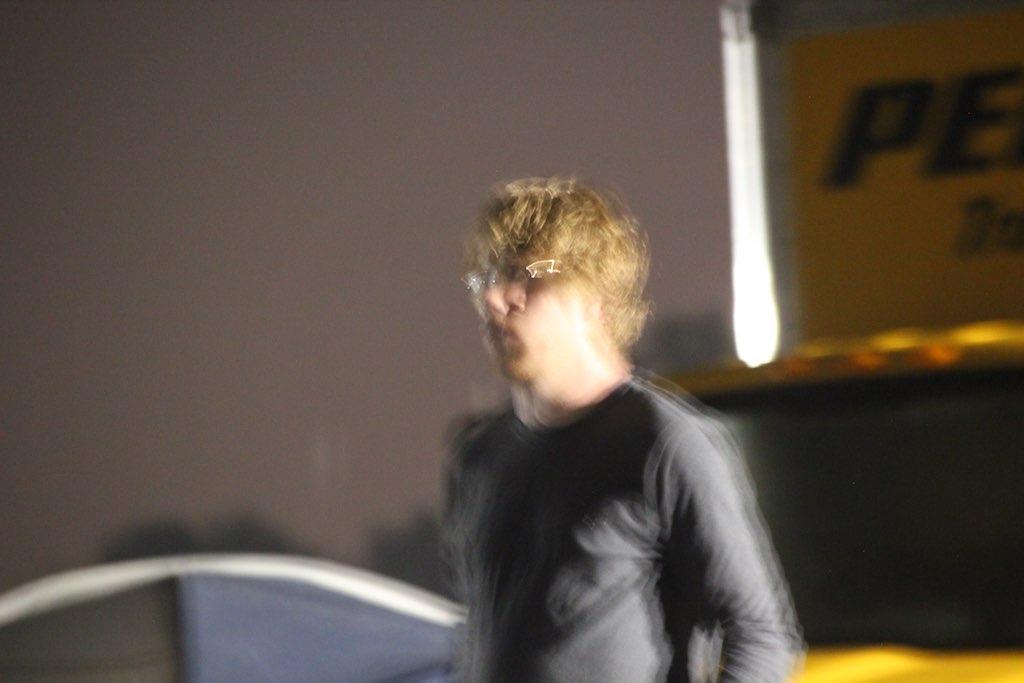In this blurred nighttime photograph, a man with shaggy, darkish blonde to reddish blonde hair, glasses, and possibly a mustache is captured mid-walk, moving from right to left while partially facing the camera. He is wearing a long-sleeve gray top that appears to cut off above the navel. To the left side of the image, there is a yellow Penske moving truck with the letters "PE" visible in bold black text, accompanied by a silver lining. The background features a light gray backdrop with some trees faintly visible. There is also a gray section below the banner and a bright, reflective area suggesting either an open door or rear edge of the truck. Additionally, there is a curved, tent-like structure with black and navy-blue colors highlighted with a white outline. The man's face is notably illuminated on the left side, possibly by a bright light source from the right. The overall image is very blurry and slightly double-exposed.